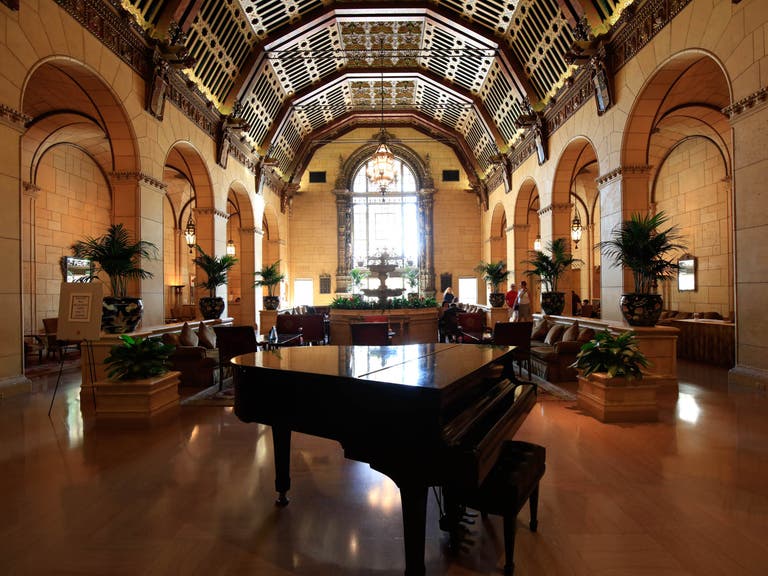The photograph captures the grand interior of what is most likely a five-star hotel lobby, exuding opulence and grandeur. Dominating the foreground is a large baby grand Steinway piano, its elegant black surface and uplifted lid designed to project music throughout the vast space. The lobby is predominantly decorated in shades of tan with darker accents, complemented by touches of green from potted plants strategically placed on ornate foyers. The hardwood floor gleams under the soft sunlight streaming in through a large, oval-topped window at the far end of the room.

The ceiling features intricate inlaid woodwork interspersed with golden vents, enhancing the lavish atmosphere, while a grand chandelier hangs majestically overhead, casting a warm glow. The background reveals a tranquil fountain close to the window, further adding to the serene ambiance. There are numerous archways—eight on either side—framing lounging chairs and sofas with plush pillows, where guests likely relax while listening to the piano music. Despite the spacious and airy feel, the furnishings suggest a high level of comfort and luxury. In the center, an elegant desk (possibly with a sculpture or vase) adds to the sophisticated décor. The overall scene is one of refined elegance, hinting at a top-tier establishment designed to provide its guests with both visual and auditory pleasures.